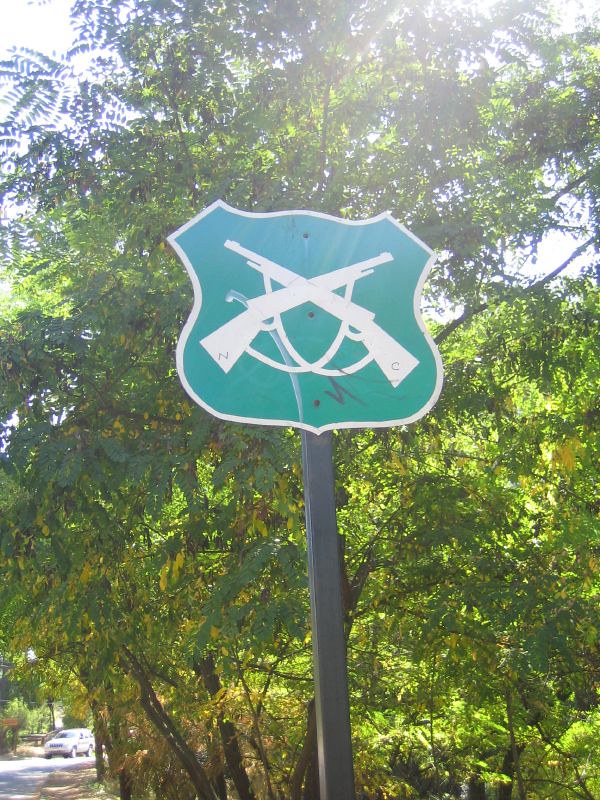This image features a distinctive sign on a residential street, characterized by its official-looking, shield-shaped design, typically associated with the Carabineros in Chile. The sign has a green background and prominently displays two white, crisscrossed rifles with shoulder straps, which are emblematic of the Carabineros. It is mounted on a square, black tubular post, standing about six to eight feet tall. The setting is a bright, sunny day with sunlight filtering through multiple trees, casting dappled shadows and creating a pleasant, suburban atmosphere. In the background, there is a mix of green trees, some with yellow blossoms, and a road with a parked car, enhancing the tranquil, residential feel of the scene. The absence of text on the sign emphasizes its simplicity and the clear conveyance of its symbolic, historical significance.